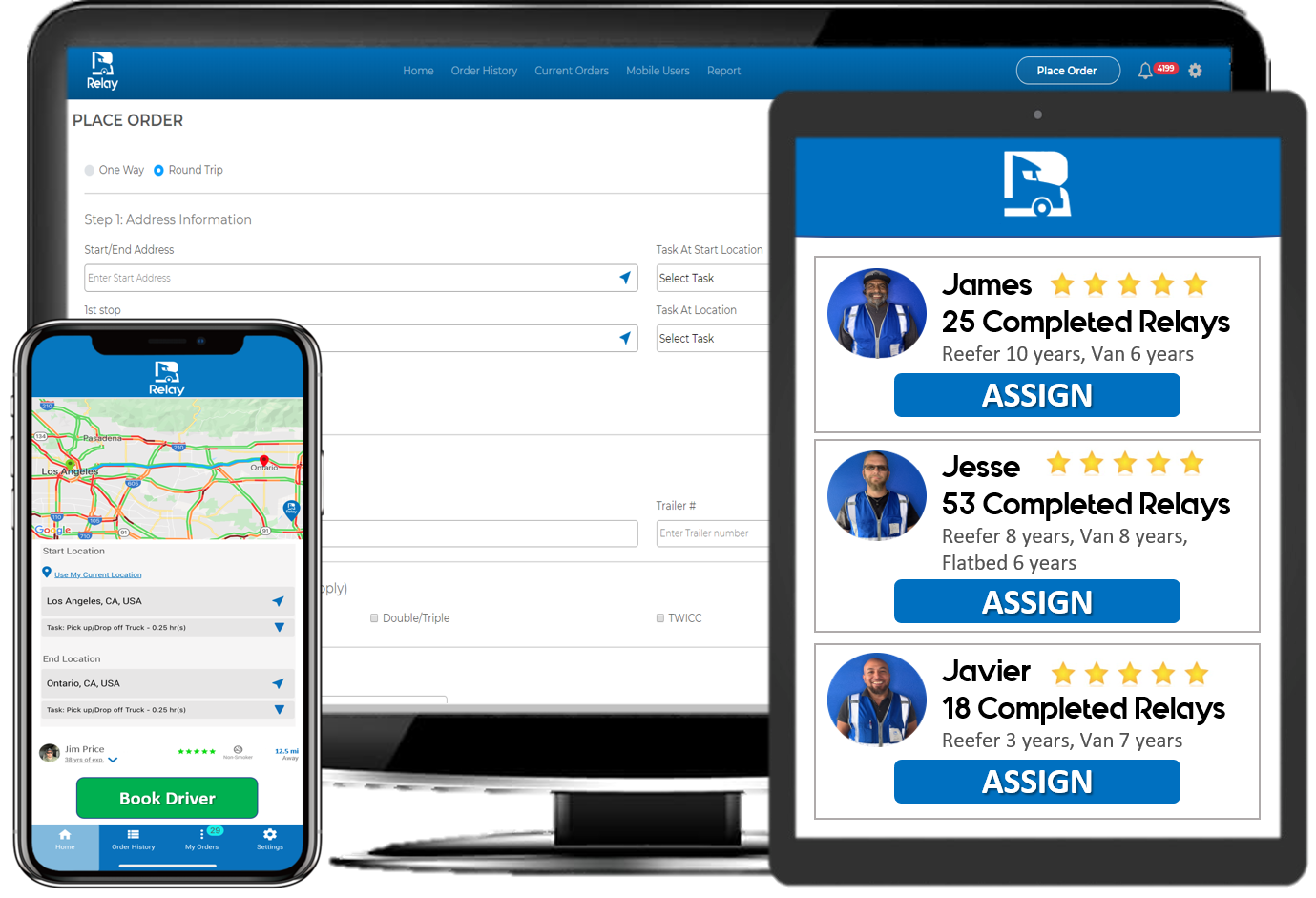This image depicts a demonstration of the Relay service interface across multiple devices, arranged around a monitor with a black frame.

In the background, the website is displayed on the monitor. It features a bright blue ribbon across the top with the word "Relay" and its blue-and-white logo in the far left corner. The screen showcases a white background with a user interface for placing an order. At the top, users can choose between a "one way" or "round trip" option, with "round trip" currently selected. Below, in the "Step One: Address Information" section, there are various fields for entering starting and ending addresses, though some of the screen is obscured by the foreground images.

In the foreground to the left, there is an image of a cell phone displaying the Relay app. The app features a blue banner at the top with the Relay logo in the center. Beneath this is a Google Map with a marked route in blue. Below the map, there are several horizontal gray boxes indicating the starting and ending locations. At the bottom is a green button labeled "Book Driver."

To the right, there's a smaller vertical rectangular screen resembling a tablet encased in a black case. This screen also displays the Relay interface with a bright blue banner at the top, showcasing the Relay logo. Below, it lists three potential drivers for selection. Each driver listing includes a profile picture, star rating, name, number of completed drives, duration of employment, and a blue "Assign" button.

Overall, this image demonstrates how Relay's service interfaces look and function across different devices, providing a cohesive and user-friendly experience tailored for users seeking transportation solutions.